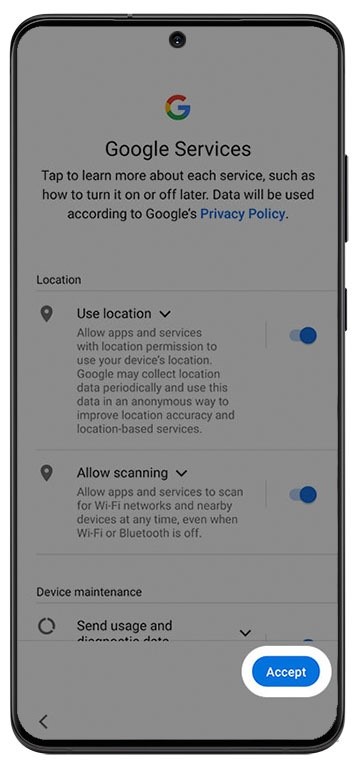The photograph captures a vertically oriented mobile phone displaying a detailed page about Google services. The phone features two black buttons on its right-hand side. Despite the slightly dim screen, the text remains legible. At the top, the iconic Google "G" logo is prominently displayed, followed by a heading that reads "Google Services."

Beneath the heading, there's a brief explanation encouraging users to tap and learn more about each service, including instructions on how to enable or disable them at a later time. This section notes that data will be managed in accordance with Google's privacy policy, with "privacy policy" highlighted in blue.

The page is segmented into distinct sections:

1. **Location**: This section starts with the subtitle "Location" and is separated by a horizontal gray bar. Below, it explains, "Use Location: Allow apps and services with location permission to use your device's location. Google may collect location data periodically and use this data in an anonymous way to improve location accuracy and location-based services." A blue toggle switch, currently enabled, is positioned to the right of this description.

2. **Scanning**: A thin gray line demarcates this section, which addresses "Allow Scanning." It states, "Allow apps and services to scan for Wi-Fi networks and nearby devices at any time, even when Wi-Fi and Bluetooth are off." This feature is also controlled by a blue toggle switch, which is in the on position.

3. **Device Maintenance and Usage**: Although brief, this section includes a conspicuous blue button labeled "Accept" in white text, indicating user consent is required to proceed.

The entire content is framed within a neat white border, giving the interface a clean and organized appearance.